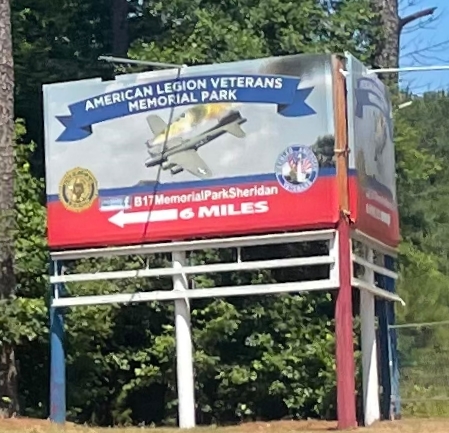In an outdoor daytime color photograph, we are presented with a detailed view of a roadside billboard. The billboard appears to form part of a larger display with two billboards positioned at a slight diagonal to each other, the right one being closer and the left receding in the background. Both billboards share a similar, if not identical, advertisement.

The billboard in focus features an olive drab B-17 bomber depicted in a downward left trajectory, with flames and black smoke pouring out from its right engine, suggesting it is in distress. Above the illustration, a blue banner spans the width of the billboard, displaying the words "American Legion Veterans Memorial Park" in bold white capital letters.

Beneath the fiery plane, another bold red rectangular section states, "B-17 Memorial Park Sheridan," also in white capital letters. Just below this, a large white arrow points to the left with accompanying text that reads, "six miles," indicating the direction and distance to the memorial park.

The billboard is supported by three poles painted in patriotic colors; the left pole is blue, the middle one is white, and the right one is red. The area surrounding the billboard includes brown grass in the foreground and trees in the background. The complementary billboard, aligned at a 90-degree angle to the right, shares the same design and message, emphasizing the cohesive promotional effort. No additional text or print is discernible in the image.